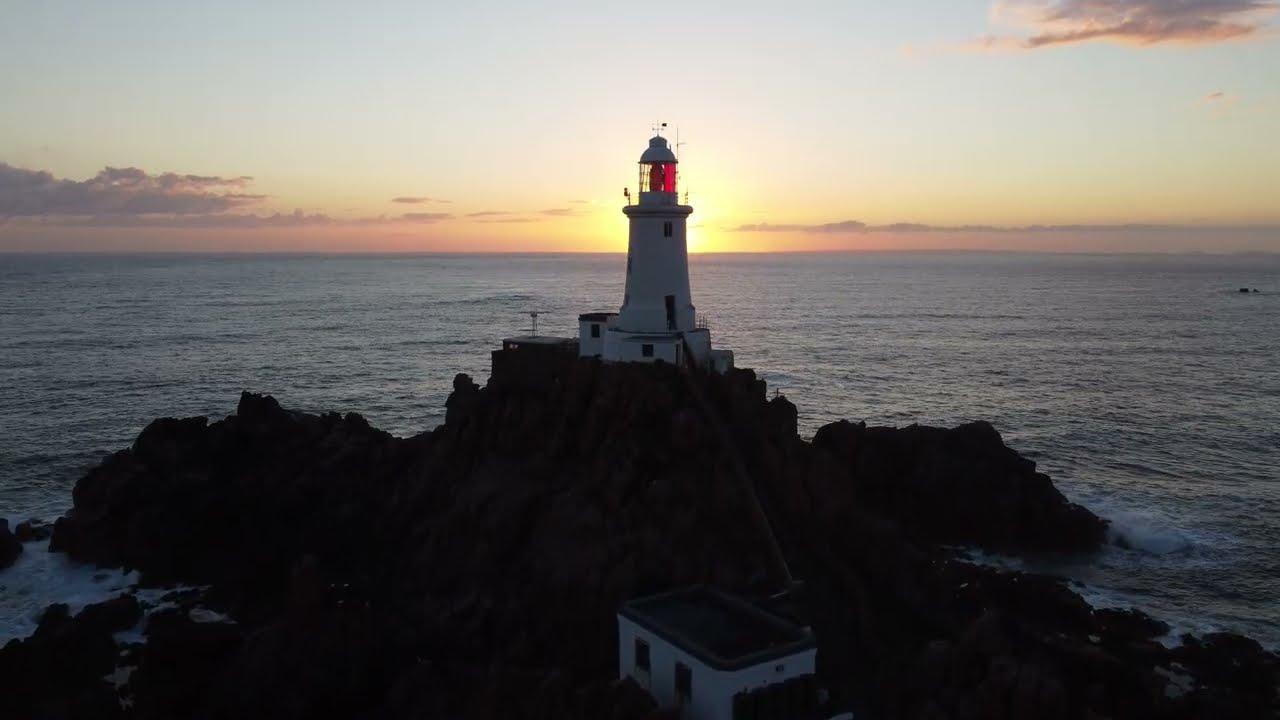This detailed landscape-oriented photograph features a white lighthouse with a black trim and a reddish dome-shaped top, centrally positioned on a small cliff overlooking a vast body of water that extends to the ocean. At the base of the cliff, a stairway with a metal railing leads up to the lighthouse entrance. Beside the lighthouse, there's a small keeper's house, characterized by two side windows and a flat black roof. The scene captures a stunning sunset or sunrise, with the sun partially obscured by the lighthouse, radiating a golden yellow and orange glow that merges into lavender and purple hues at the edges of the sky. The sky is adorned with a few scattered clouds, contributing to the picturesque outdoor setting. The overall atmosphere is serene, with the vibrant colors contrasting the darker tones in the foreground.